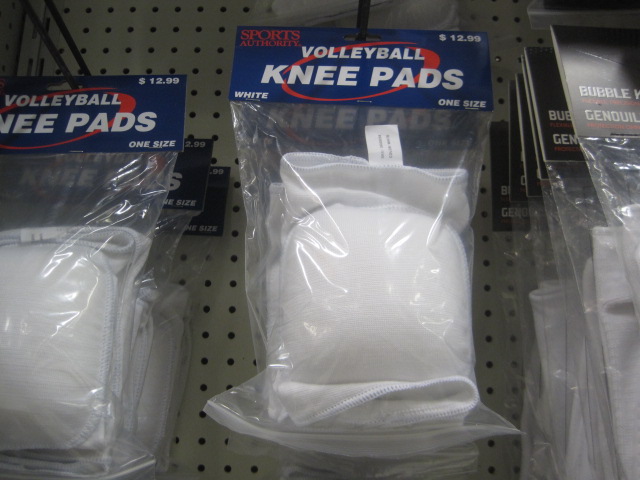This image captures a retail display within a sporting goods store, featuring prominently packaged white volleyball knee pads. The knee pads, priced at $12.99, are from the Sports Authority and are clearly labeled "One Size." They are neatly hung on black hooks affixed to a white, cream-colored pegboard background, which is dotted with holes typical of such retail setups. The packaging is transparent, allowing the white knee pads to be fully visible. Adjacent to the main row of knee pads, another row of similar-looking knee pads is partially captured but not fully legible, indicating more options available. The setting is clean and straightforward, typical of indoor store environments, and every detail—from the colors to the price and branding—is clearly laid out, making the knee pads noticeable to potential buyers.